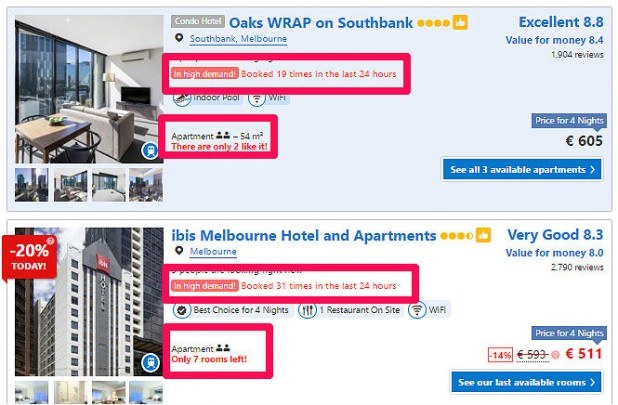Screenshot of a website's selection page for accommodations:

At the top, there is a light blue rectangle bordered with a black line. In the upper center of this rectangle, "Oaks Wrap on South Bank" is displayed in blue font. To the right, four yellow circles and a yellow square with a white thumbs-up icon are visible. Adjacent to these icons, in blue font, it reads: "Excellent 8.8. Value for money 8.4. 1,904 reviews."

Below the blue rectangle, "South Bank Melbourne" is written. Surrounding this text is a red highlighted square containing the message: "In High Demand. Booked 19 times in 24 hours." Beneath this, another red square states: "Apartment 54M. There are only two like it." Further down, it shows the price: "£605 per night," and an option to "See all 3 available apartments."

To the far left of this section, there are pictures of the apartment's interior, which appears to be a typical apartment setting.

Below this listing, there's another selection for "Ibis Melbourne Hotel and Apartments."